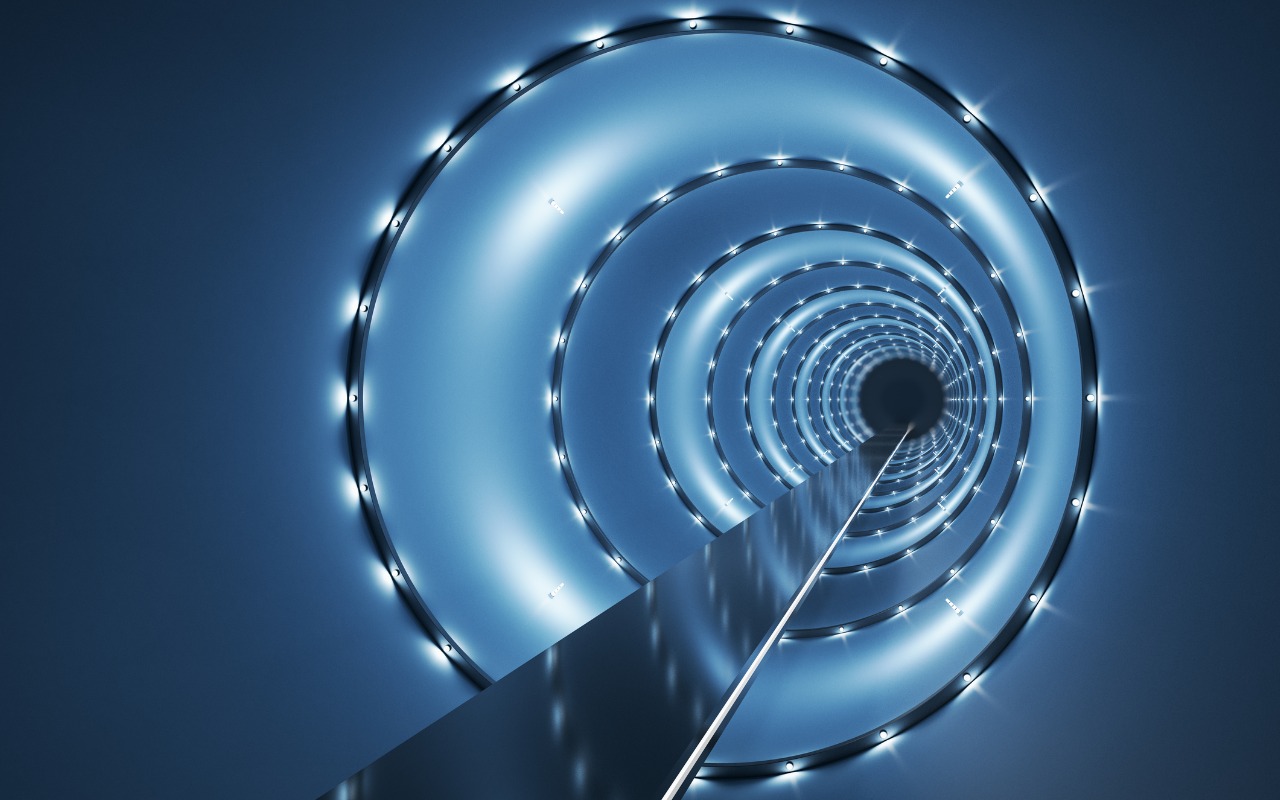The image depicts a mesmerizing, futuristic scene featuring a spiral tunnel with a blue tinge that transitions from darker around the edges to lighter in the center. The focal point is a series of concentric black circles illuminated by bright white lights at regular intervals, creating an optical illusion of diminishing into infinity. Alternating with these circles are slightly white bands, each adorned with four small lights, enhancing the tunnel's depth and complexity.

At the center, a reflective, slightly matte, silvery walkway stretches towards the distant darkness, bordered on the right by a continuous bright white light. This path appears to lead into an enigmatic black void with a faint gray outline, giving an impression of an endless journey. The outer structure of the tunnel is composed of darker gray metal, creating a cylinder-within-a-cylinder effect. The reflection on top of the walkway distorts the concentric circles and lights, adding to the surreal atmosphere. The overall color palette includes shades of black, blue, light blue, gray, and white, contributing to the otherworldly and immersive visual experience.